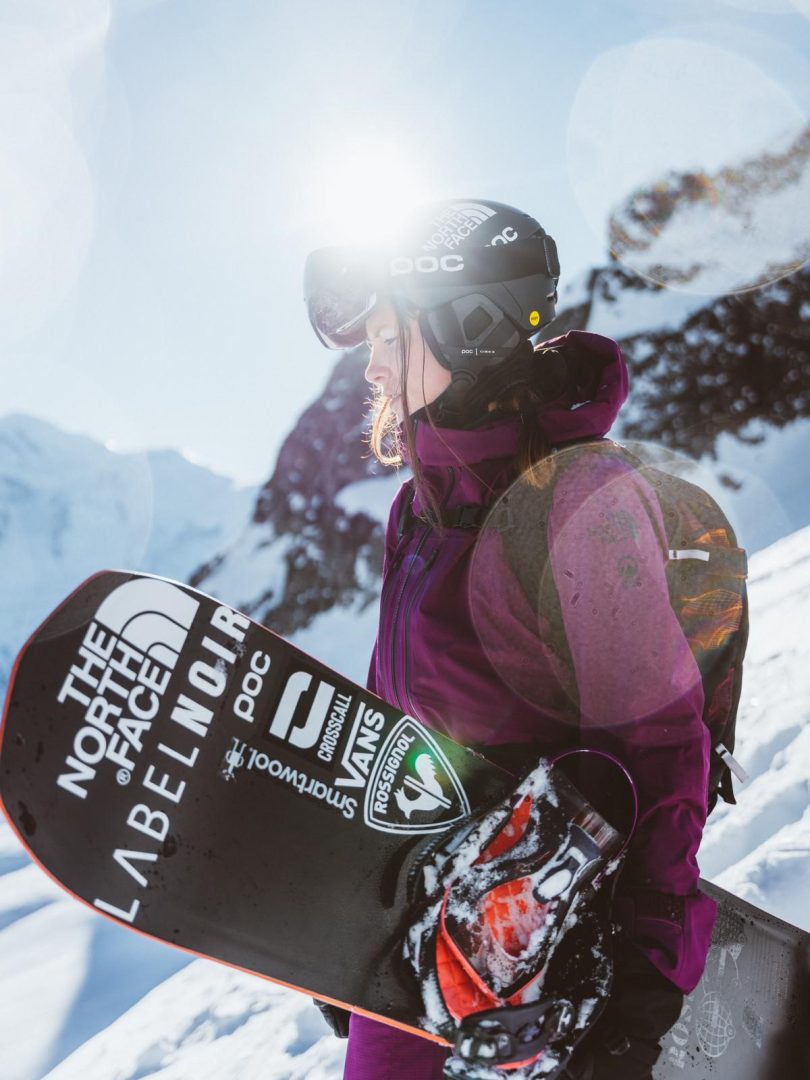In this outdoor daytime photograph, a female snowboarder stands on a snowy mountain under a sunny sky, with the sun shining brightly behind her head. She is wearing a black helmet with black goggles, a purple jacket paired with purple snow pants, and black gloves. Slung over her shoulders is an orange and black backpack. Her long brown hair is braided into a short braid. She holds a sleek black snowboard, adorned with white and orange foot clamps and encircled by an orange border. The snowboard features various logos including The North Face, Vans, and others. The vivid brightness of the sun casts a radiant glow over her helmet, partially obscuring the top of her head from view. The snow-covered, rocky mountain terrain stretches out behind her, highlighting the serene yet adventurous setting.